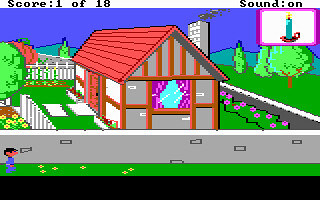This image appears to be a screenshot from an retro video game with 8-bit graphics, likely from the 80s or 90s. The primary focus is a house with a primitive yet charming design, featuring a red roof, gray or white walls, a white picket fence, and a white brick chimney emitting smoke. The front of the house is marked by an orange or brown door, with blue windows adorned by purple or pink drapes. The house is surrounded by a colorful garden with green bushes, trees, and various flowers in shades of purple, yellow, and pink. A stone wall or fence encloses the garden, through which a green walkway leads up to the house. In the bottom section of the image, a small person or child with black hair, dressed in blue, is seen walking outside the stone fence.

Above the house, the top section of the screen displays "Score: 1 of 18" on the left and "Sound: On" on the right. There is also a small purple-bordered white box in the upper right corner, containing an image of a blue candle on a pink plate. The scene is set against a bright blue sky with some distant hills, contributing to the idyllic, nostalgic vibe of this game screenshot.